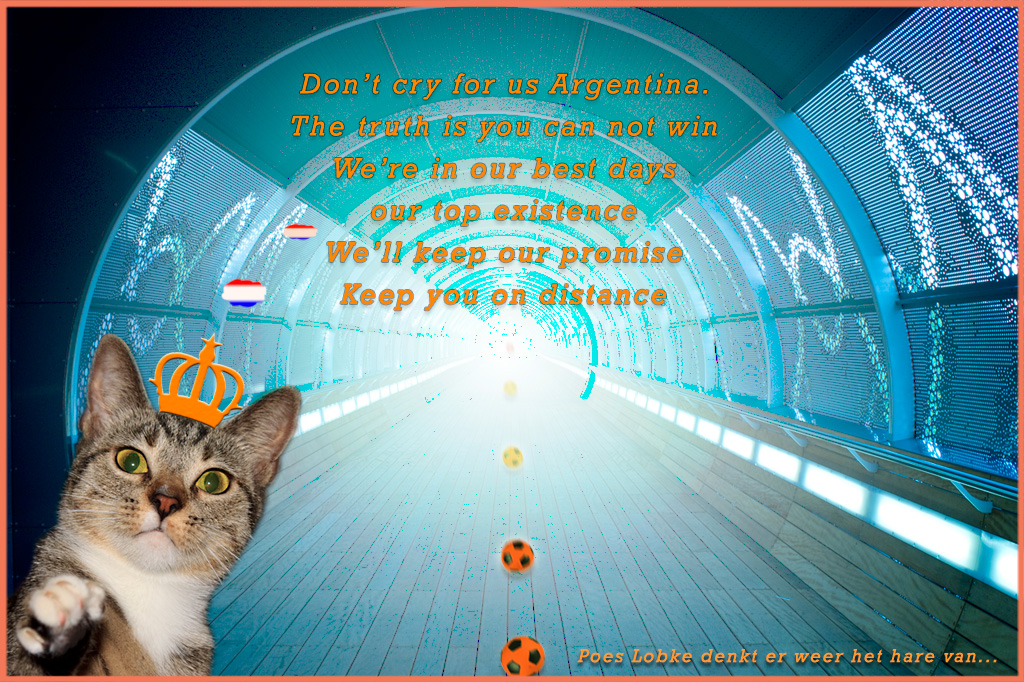In this digitally generated, landscape-oriented image, a light blue circular tunnel extends into the horizon, creating a bright central area against darker corners with blue arcs overhead. Along the wood-plank floor of the tunnel, a row of orange and black soccer balls recedes into the distance. Decorating the sides are twinkling lights and abstract white formations. In the bottom left corner, a superimposed photograph of a gray and black striped cat gazes at the viewer, wearing an illustrated orange crown atop its head. Adjacent to the crown, two red, white, and blue colored designs are seen, adding a flag-like element. At the top center of the image, in orange text, is the quote: "Don't cry for us Argentina. The truth is you cannot win. We're in our best days, our top existence. We'll keep our promise, keep you on distance."